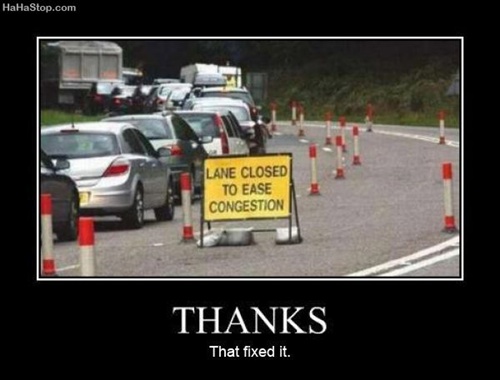The image is a meme featuring a traffic scene. At the top left-hand corner, white text reads "hahastop.com" on a black border. Below the traffic image, the black border continues with white text stating, "THANKS, THAT FIXED IT." The main picture shows a roadway with two lanes. The left lane is congested with cars lined up in traffic, including a black car at the back, a silver car in front of it, a greenish car, a white car, and several darker-colored cars that are less distinct. There is also a large gray truck that appears designed for hauling materials. The right lane is closed, separated by red and white construction cones. The closure is marked by a yellow sign with black text that reads, "LANE CLOSED TO EASE CONGESTION," supported by sandbags. The road curves and features white lining. The setting includes grassy hills and trees in the background, indicating the scene is outdoors during daylight hours. The clear lighting highlights the greenery and overall clarity of the image.